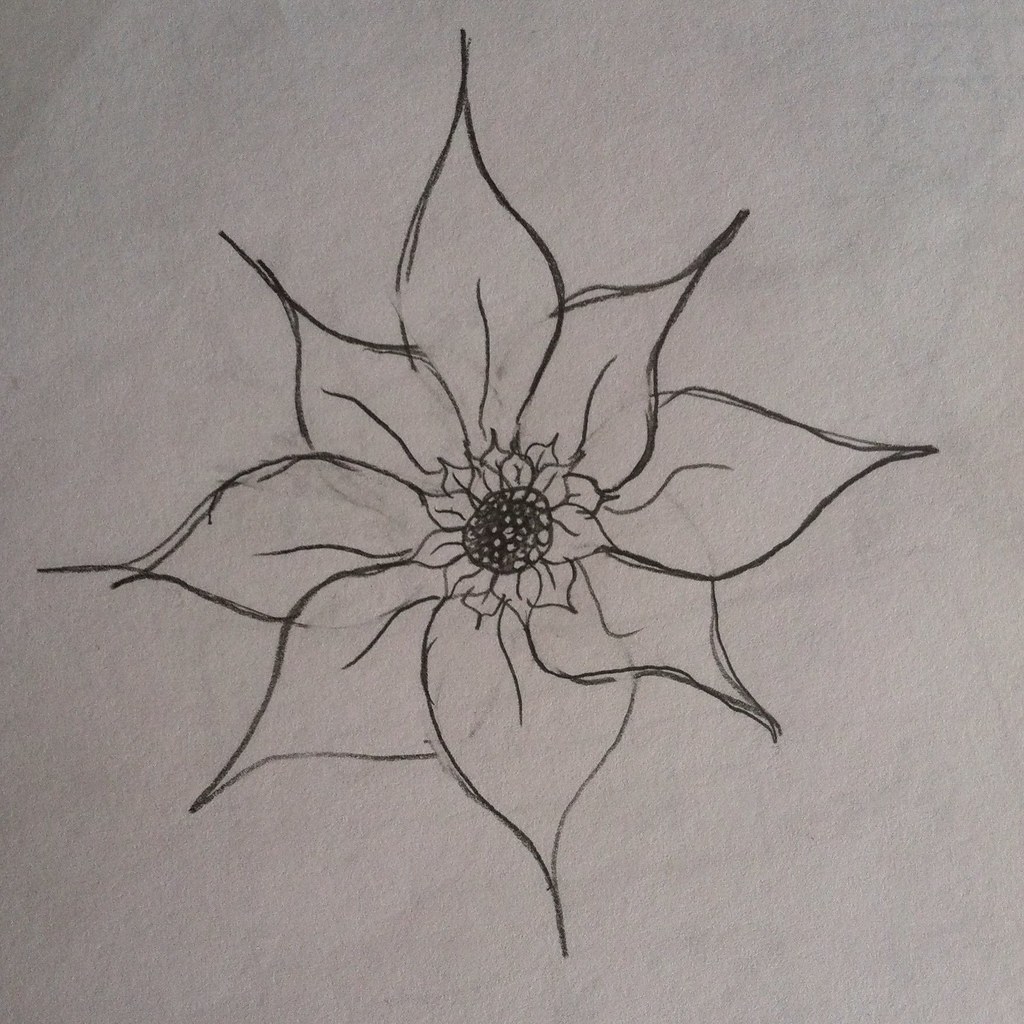A detailed, hand-drawn illustration of a flower, likely a poinsettia or lotus, is centered on a white, textured piece of paper. The flower, which appears to be sketched with either pen, ink, or a dark lead pencil, exhibits eight petals extended outward in a symmetrical pattern. Each petal is broader and rounder near the center, tapering to a sharp, almost thin point at the edges. They feature central veins, adding to the intricate detail. The center of the flower is decorated with a black and white speckled dot, surrounded by tiny overlapping petals, each defined with delicate lines. The high-quality paper, despite some subtle shadows giving it a slightly gray tone, highlights the skill of the artist, suggesting this is a photograph or scan of the original drawing. The piece does not have any visible shadows or an artist's signature, emphasizing its illustrative quality and the artist's attention to detail.